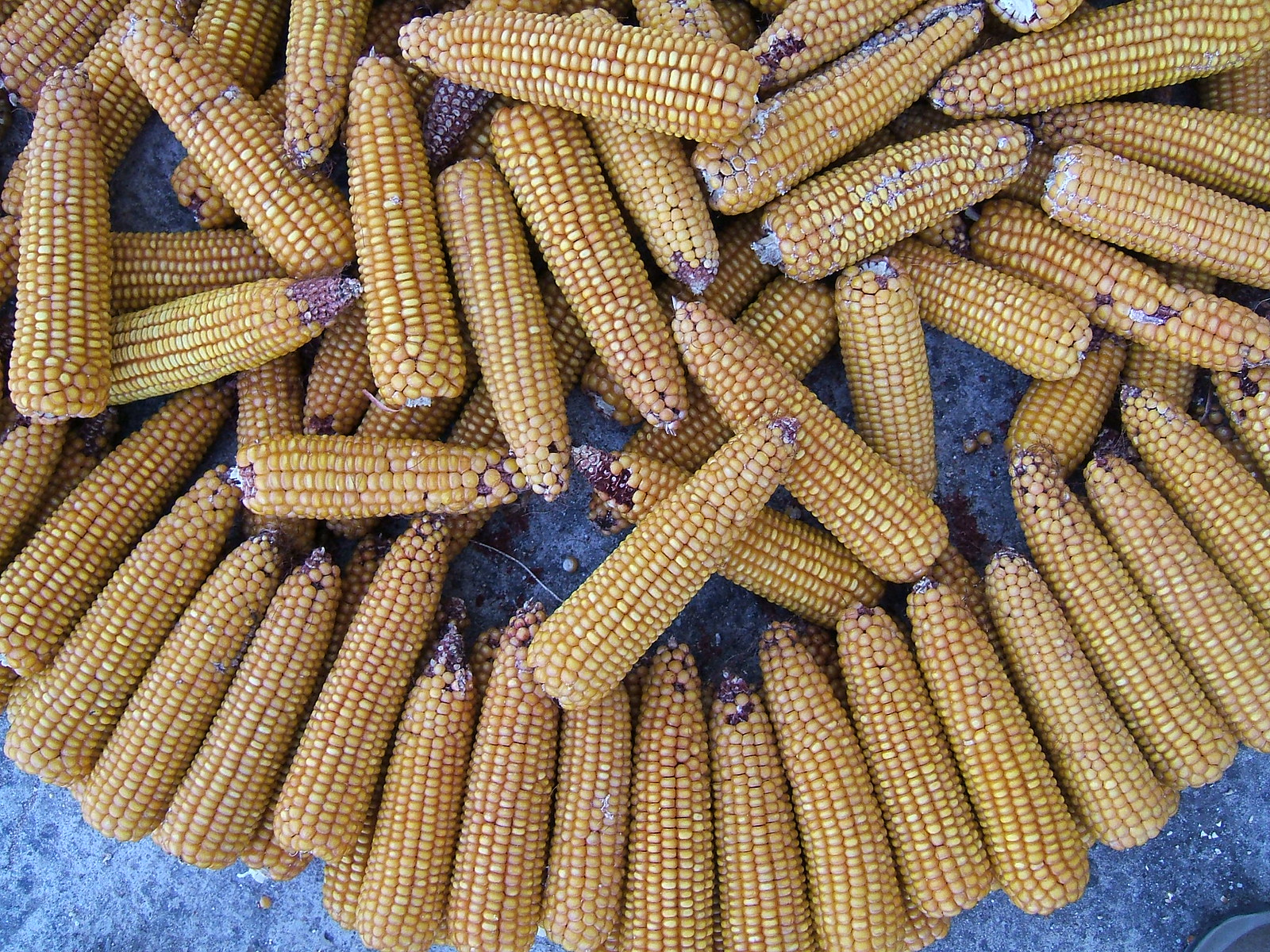This image features an overhead view of several ears of corn arranged inside a large container with a grayish-blue hue. The container, resembling a pot or a large bowl, serves as the backdrop for the corn. The ears of corn, which are intended for animals such as deer or squirrels rather than for human consumption, exhibit a dull yellow color with various imperfections, including browned and gray sections, blackened tips, and missing kernels.

The overall configuration of the corn is a striking contrast between order and chaos. Around the perimeter, the ears are meticulously aligned to form a ring-like circle, with their larger bud parts facing outward and smaller ends pointing inward. In the center, however, the ears are haphazardly piled, extending in every direction without a discernible pattern. This chaotic pile includes ears with noticeable white spots and significant kernel loss.

The ground beneath the container is ambiguous, appearing either as blue table-like surface with black and white flecks or possibly a road or concrete dirt ground. The texture and color details of both the container and the corn enhance the rustic and utilitarian appearance of the scene, emphasizing the corn's purpose as animal feed.